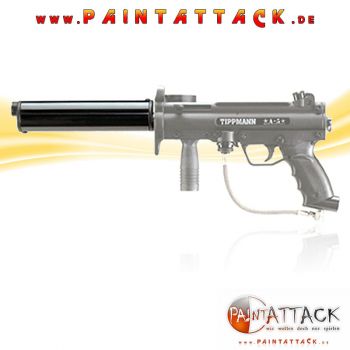The image showcases a semi-realistic paintball gun, resembling a pistol, in a detailed side profile. The main body, including the handle and chamber, is gray, while the long barrel extending to the left is black. White letters on the gun spell out "Tippmann." The backdrop is predominantly white, contrasted by a gold swirl that threads from left to right behind the gun. At the top of the image, a web address, www.paintattack.de, stretches across in red letters transitioning from yellow at the top to red at the bottom. In the bottom right corner, a logo reading "Paint Attack" is displayed, with the website URL repeated below in smaller text. The setting is brightly lit, ensuring clear visibility of all elements.